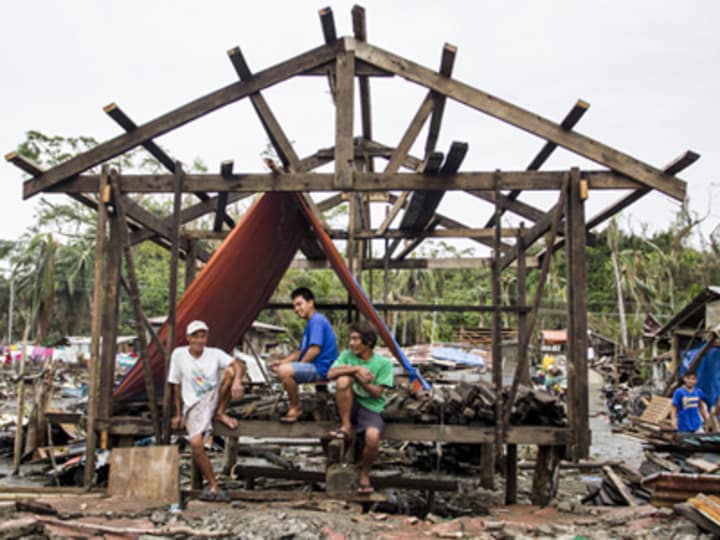The image depicts a blurred photograph of the skeletal wooden frame of what appears to be a house amidst the aftermath of a natural disaster, possibly a fire or storm, situated in a tropical environment. The frame, strewn with debris and wood, suggests a scene from Southeast Asia—potentially Indonesia, the Philippines, or Burma. Three men of Southeast Asian descent, identifiable by their light brown skin and attire, are seated on the edge of the floor structure. The man on the left wears a white t-shirt with a design and a white baseball cap, the central figure is dressed in a blue t-shirt and blue shorts with flip-flops, and the third man in a bright green t-shirt looks off to his right, our left. They are resting amidst the remnants of a structure with a makeshift shelter—a large tarp or canvas draped over a beam—possibly indicating temporary refuge against the elements. The background shows dense, jungle-like greenery, emphasizing the tropical setting, while the surrounding area is littered with debris, evoking a sense of destruction and disrepair. The overall scene suggests a community grappling with significant devastation, the precise cause of which remains unclear.